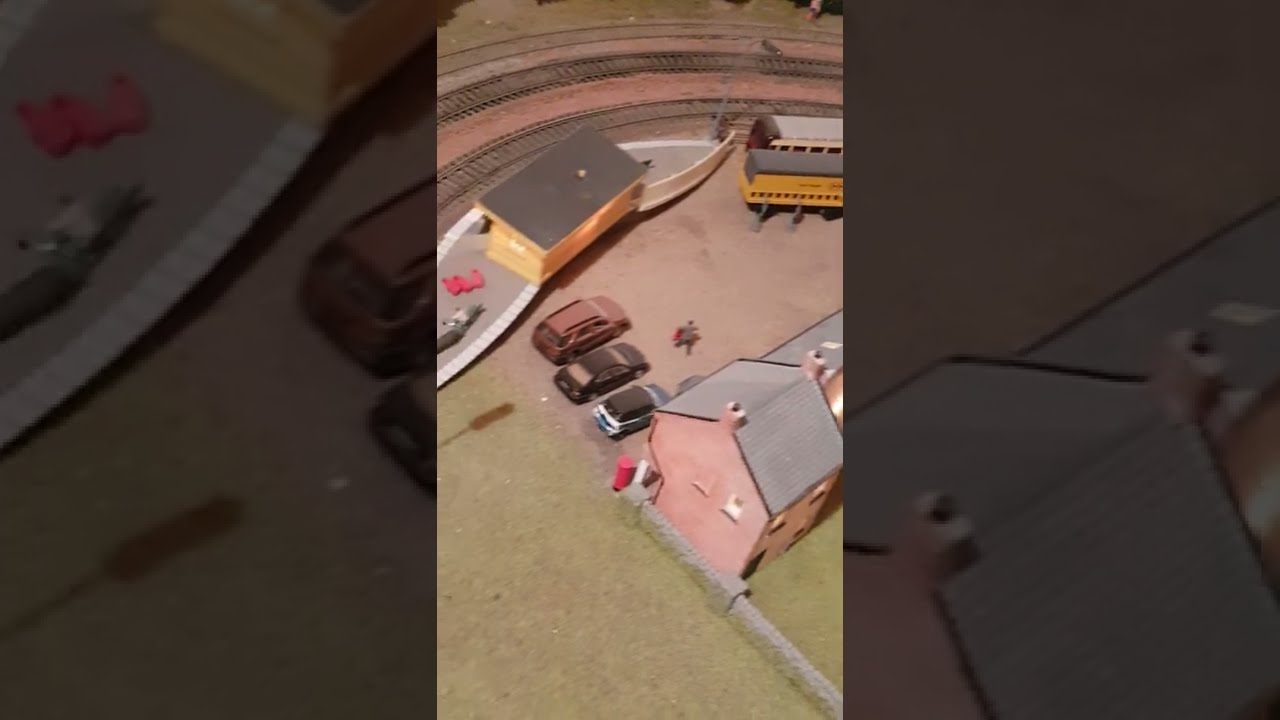The image is a horizontal rectangle divided into three equal sections. The left and right sections are darker, while the middle section is well-lit. The overall scene appears to depict a model train set with detailed surroundings.

In the left section, a darkened view shows a street bordered on the right by a wall. The street has vehicles that appear cut off towards their rear, ascending slightly to the right. The wall on the left borders some indistinct images, one pink and one gray.

The middle section, which is brightly lit, features an aerial view of a model house with a grassy area on one side and a parking area on the other. The parking area contains three vehicles, and nearby, a second building enclosed by what looks like a white stone fence sits close to some railroad tracks. These tracks curve at the top part of the image. Nearby are a couple of railroad cars stationed off the tracks. Various colors like green, brick red, gray, black, white, yellow, and earthy browns enhance the detailed scenery, which includes small model cars and other miniature elements.

In the right section, another darkened view shows just the rooftops of two buildings at the bottom of the image, hinting at more peripheral details of the model scene not fully visible due to lighting and cropping.

Overall, the photo appears to be a low-quality vertical shot from a phone camera, capturing a model train set with intricate details such as tracks, buildings, cars, and train stations, adding to the charm and realism of the miniature world.